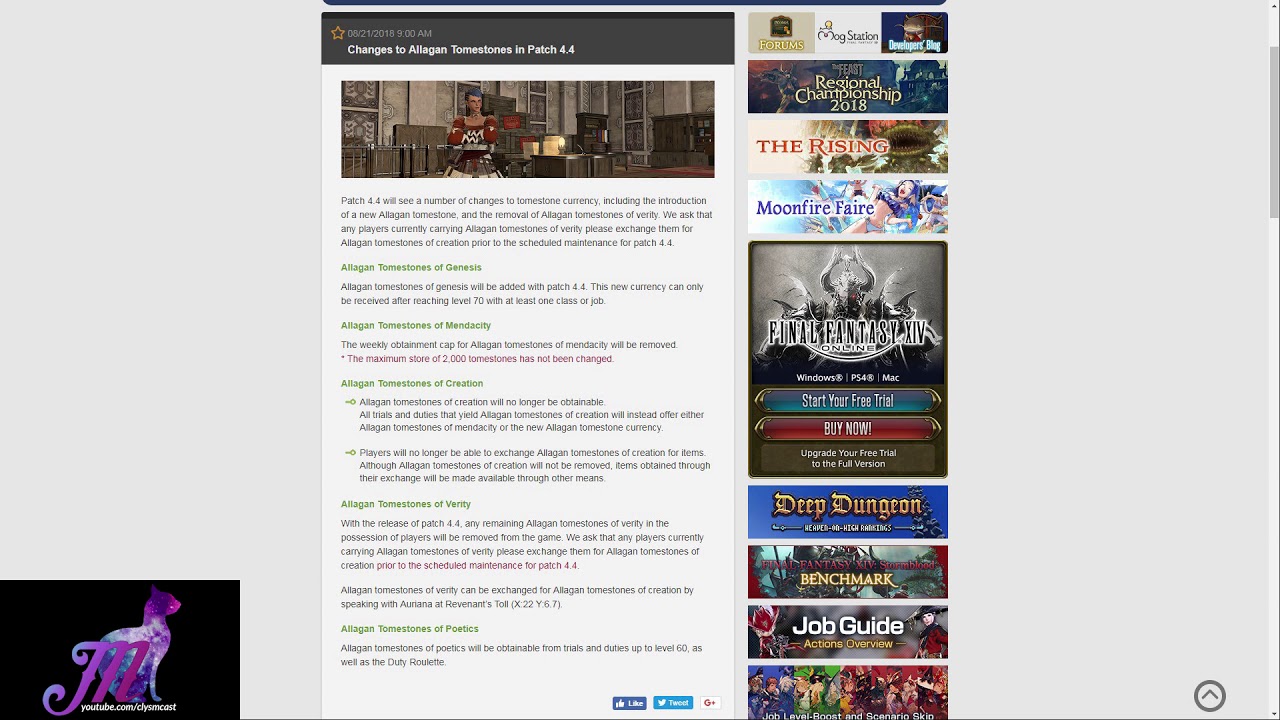This screenshot features a comprehensive list of twelve video games, each sequentially numbered from 1 to 10. The list is accompanied by a detailed game description spanning eight paragraphs. The visual design includes a distinctive black box at the bottom, adorned with a gradient color showcasing the letter "M," which transitions into the image of a cat. Additionally, there are options to like and share the content, suggesting that this image might be from a blog or another online platform where users can interact with the post.